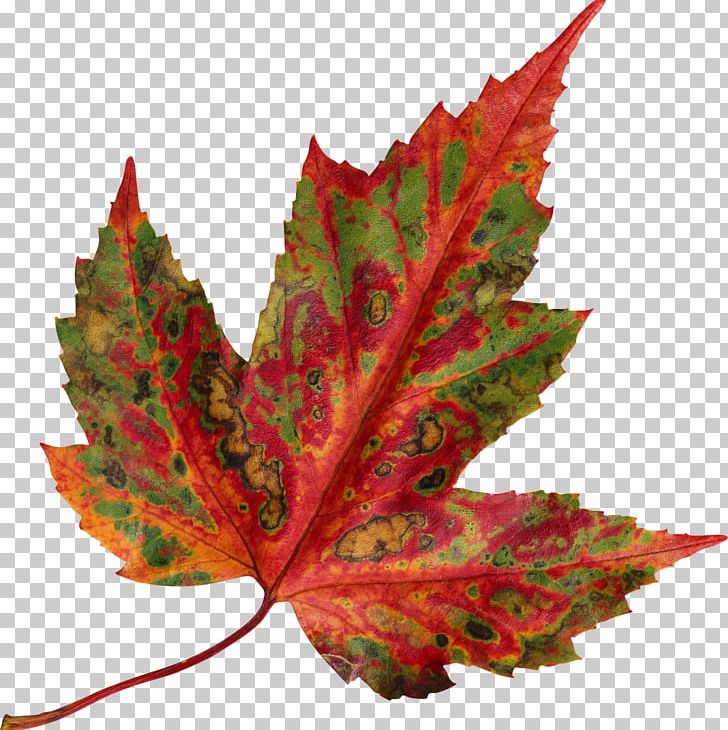In this captivating image, a large, maple-like leaf dominates the frame, perfectly centered against a translucent background with a gray and white checkerboard pattern. The leaf, in an autumnal state, showcases a dazzling array of colors: vibrant red, orange, green, and scattered yellow spots, some of which are edged in black, indicating decay. The leaf is uniquely composed of three ridged parts or spikes, each connected by a prominent, central vein that runs through the leaf and connects at the base to a brown and red stem. The contrast of the bright colors, the intricate patterns, and the checking condition of the leaf suggests a psychedelic yet natural artwork, making it visually striking and vivid, suitable for digital use or web integration due to the image's transparent background.